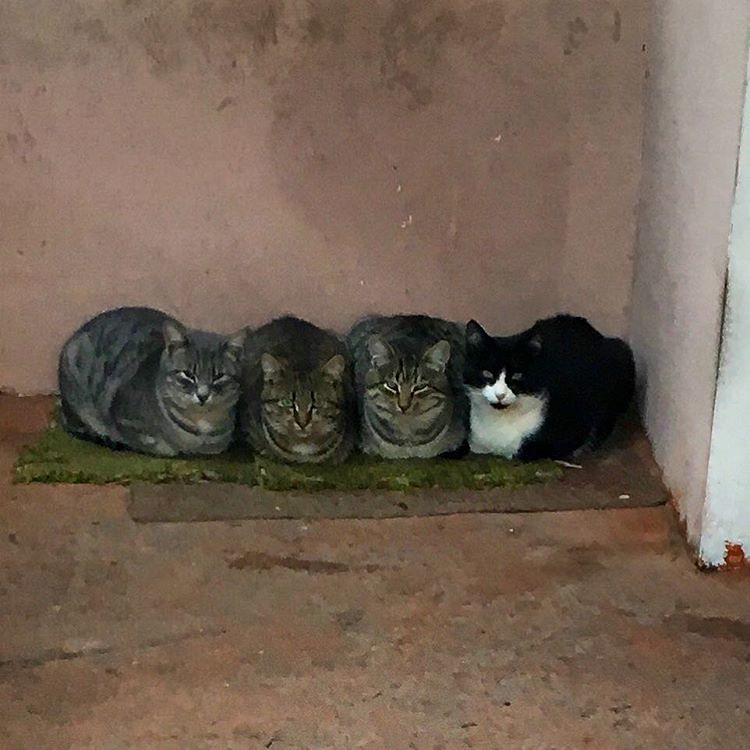In this photograph, four cats are seen resting side by side outside in the corner of a building, against a worn, light-colored wall with visible patches where the paint has come off. The cats are reclining on an old, layered mat, with the topmost mat appearing green and resembling a piece of artificial grass. The ground beneath the mat looks dirty and weathered. The positioning and appearance of the cats are distinct: three of them, located on the left, are tiger-striped with similar brown and gray markings and green eyes, suggesting they might be of the same breed. The fourth cat, on the far right, stands out with its black and white coloring, featuring a black body contrasted by white on its chest and the lower half of its face. The picture captures a front-view perspective, showcasing the cats relaxing closely together and gazing towards the camera.